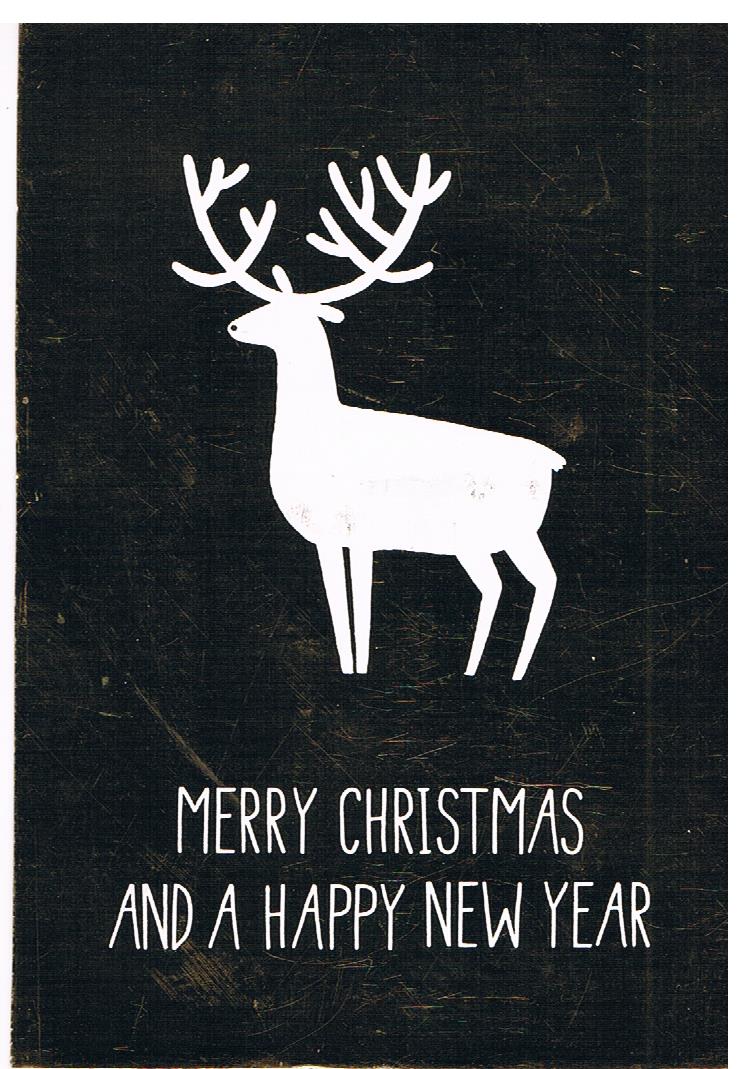The image features a minimalist Christmas card or social media graphic with a textured background resembling aged, scratched black metal or fabric. The central figure is a simplistic, solid white cartoon illustration of a reindeer facing left, characterized by a small black dot for a nose, U-shaped antlers extending from its head, rounded ears, and together front legs. The reindeer's long, rounded body, small tail, and distinct hind legs complete the figure. Below the reindeer, in thin, white text, is the holiday greeting: "Merry Christmas and a Happy New Year." The overall dark gray or black background is heavily marked with white scratches and scuffs, contributing to the worn, vintage aesthetic.